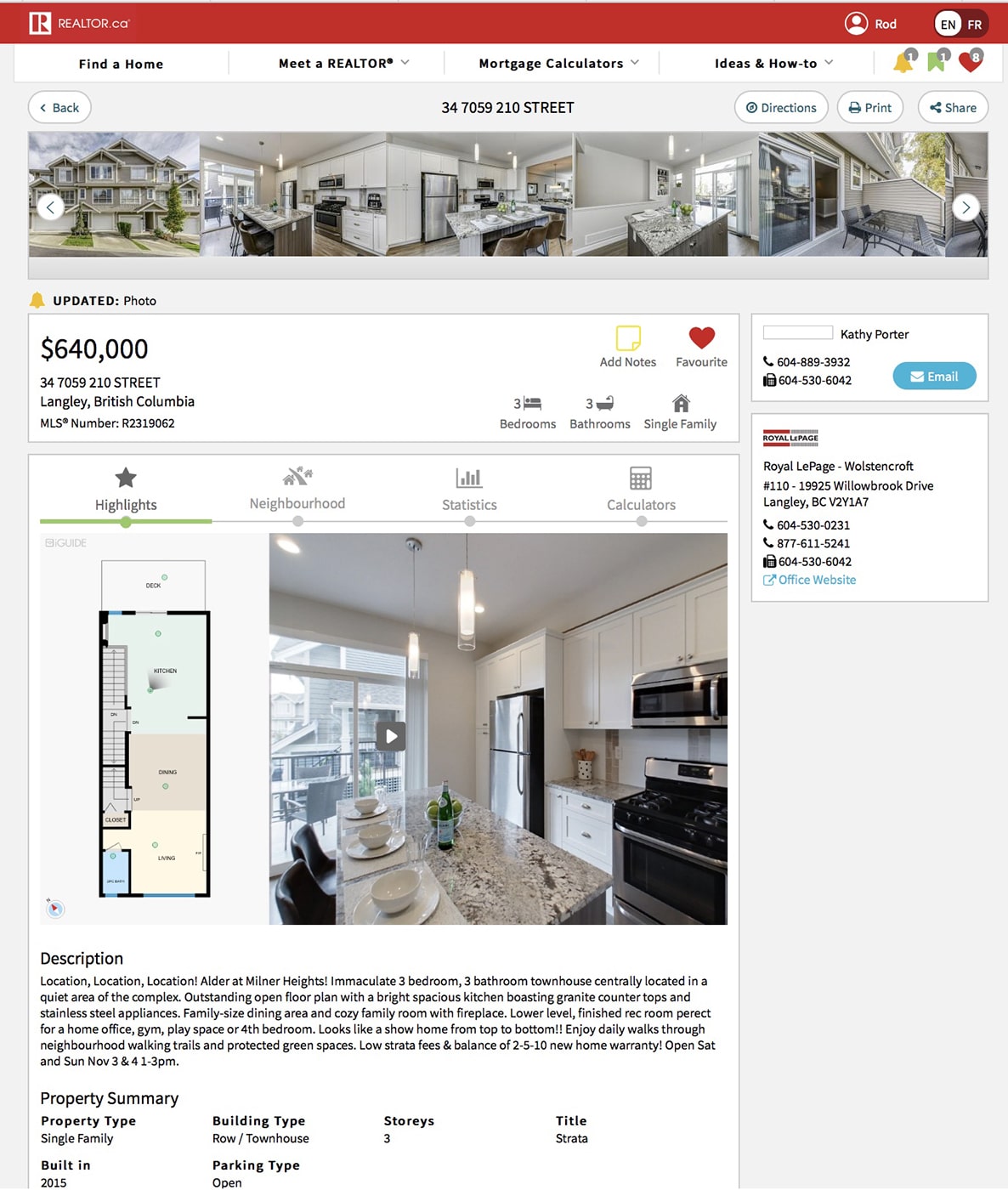This image features a webpage from realtor.com, showcasing a detailed property listing. At the top of the page, users can navigate through options such as "Find a Home," "Meet a Realtor," "Mortgage Calculations," and "How-To Ideas." Notification, bookmark, and heart icons are prominently displayed for user convenience. The main section displays various images of a house, which can be browsed using arrows on either end. 

The highlighted property is located in Langley, British Columbia, and is listed for $640,000. It includes an overview of the house's key features, including a detailed floor plan, a description of the property, and images, such as one of the kitchen.

Key property details are listed:
- Property Type: Single Family
- Building Type: Row Townhouse
- Year Built: 2015
- Parking Type: Open
- Storage: 3 units
- Title: Strata

The realtor's information is also provided, with a contact name that is either Kathy or Kelly, along with her phone number, fax number, and a blue button for emailing her. Additional contact details for Royal LaPage include two more phone numbers and a fax number, along with a link to the official website. 

Users can also access information about the neighborhood, including statistics and various calculations related to the property.